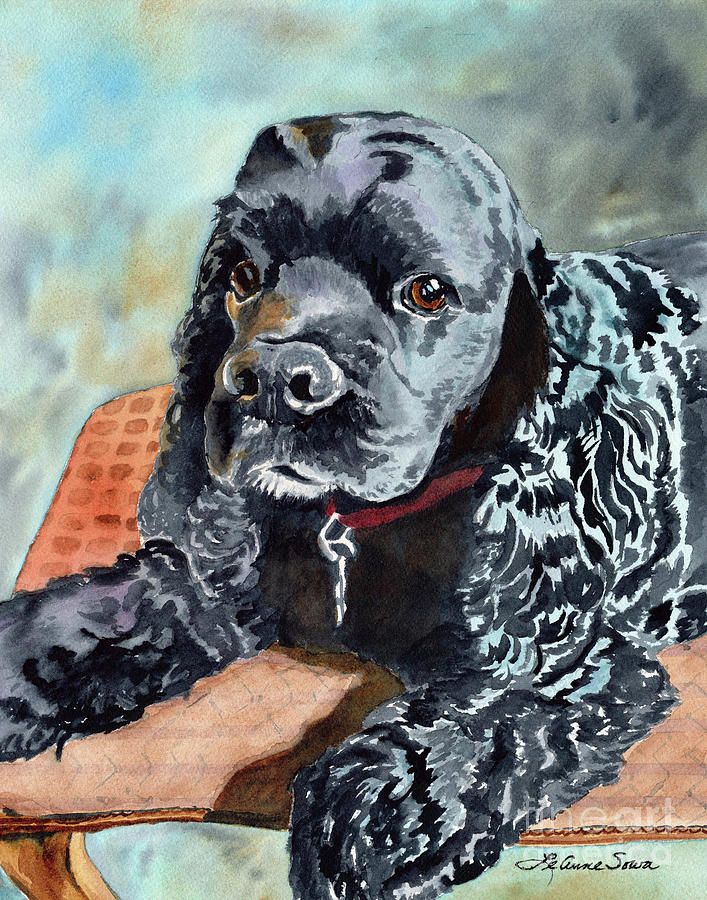This image is a detailed watercolor painting of a black spaniel-like puppy with long floppy ears and brown eyes, sitting on a stool. The dog is facing forward but slightly to the left, giving the impression that it is looking at the camera. It has a red collar with a silver clasp and a small, sideways-turned tag. The canine's left paw is visible on the right side of the image, while its right paw extends off the canvas to the left. It seems to be perched on an orangish-red cushion with a faint checkerboard pattern, supported by a visible wooden leg in the bottom left corner.

The background of the painting is a blend of blue and gray hues, creating a soft and blurred effect that contrasts with the dark fur of the puppy. In the upper right-hand corner, the color transitions into darker patches of black, enhancing the overall depth of the piece. At the bottom right-hand corner, the artist's signature appears in black cursive letters, though it is partially obscured by a transparent watermark with white lettering.

Overall, the painting captures a tender and serene moment, with the detailed texture of the dog's fur and the subtly colored background contributing to a warm, inviting atmosphere.